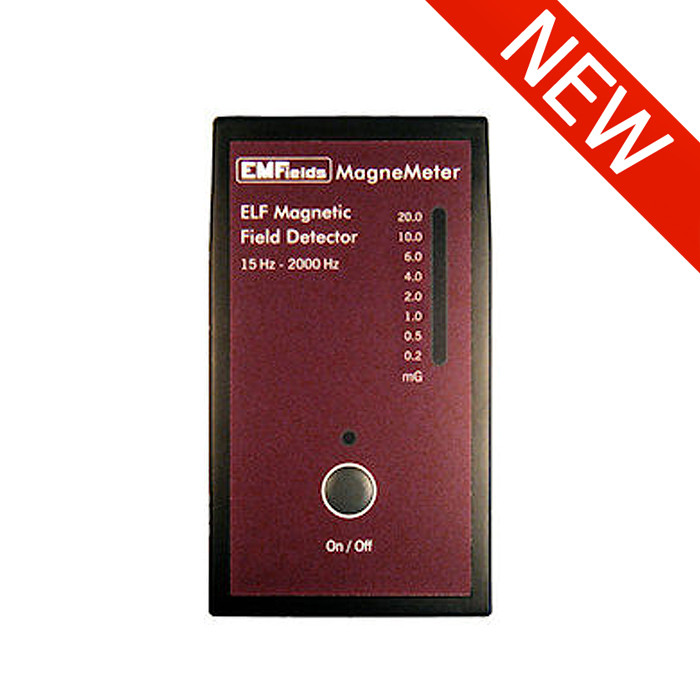The image prominently features a single object, well-centered and zoomed in for clear visibility, set against a completely white background. In the upper right corner, a medium red diagonal ribbon marked with "New" in white letters emphasizes the advertisement nature of the image. The object is a tall, rectangular device outlined in black with a maroon center, featuring the text "EM Fields Magnimeter, ELF Magnetic Field Detector, 15 Hz to 2000 Hz" in white letters. On its right side, the device has a tall oval meter labeled "MG" at the bottom, with numbers ranging from 0.2 to 20, increasing upwards. At the bottom of the device, there is a circular black on-off switch. The colors present in the image are white, red, maroon, and black, enhancing the advertisement’s visual appeal and clarity.